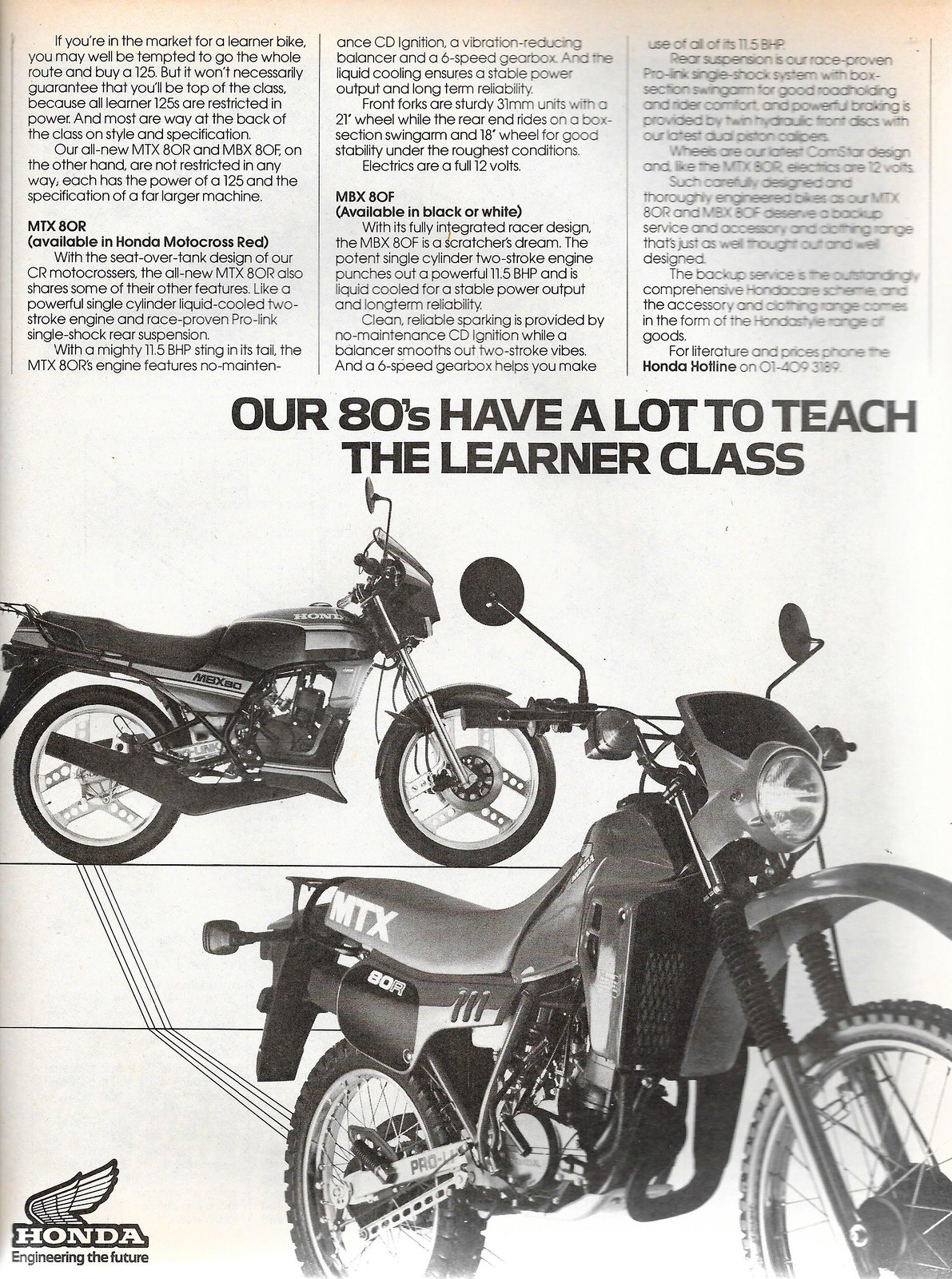This vintage advertisement, likely from a 1980s motorcycle magazine, showcases two Honda motorcycles in a detailed black-and-white image, though the top of the page is tinged yellow with age. The ad prominently features the Honda logo and the tagline "Engineering the Future" in the bottom left corner. Centered above the two motorcycle images, the headline reads, "Our 80s have a lot to teach the learner class." 

The motorcycles are distinct models: the MTX-80R, available in Honda motocross red, and the MBX-80F, offered in black or white. The MTX-80R is an enduro bike that is versatile for both street and dirt riding, sporting high handlebars above the gas tank, a higher seat, and an elevated exhaust system. In contrast, the MBX-80F is a street bike characterized by lower handlebars with a small windshield, star-shaped six-spoke rims, and exhaust pipes running beneath the foot pegs. 

The text emphasizes the superior power and specifications of these models compared to restricted learner 125cc bikes. Finally, the ad invites potential buyers to call a provided phone number for more information, a quaint touch from an era before digital communication dominated.